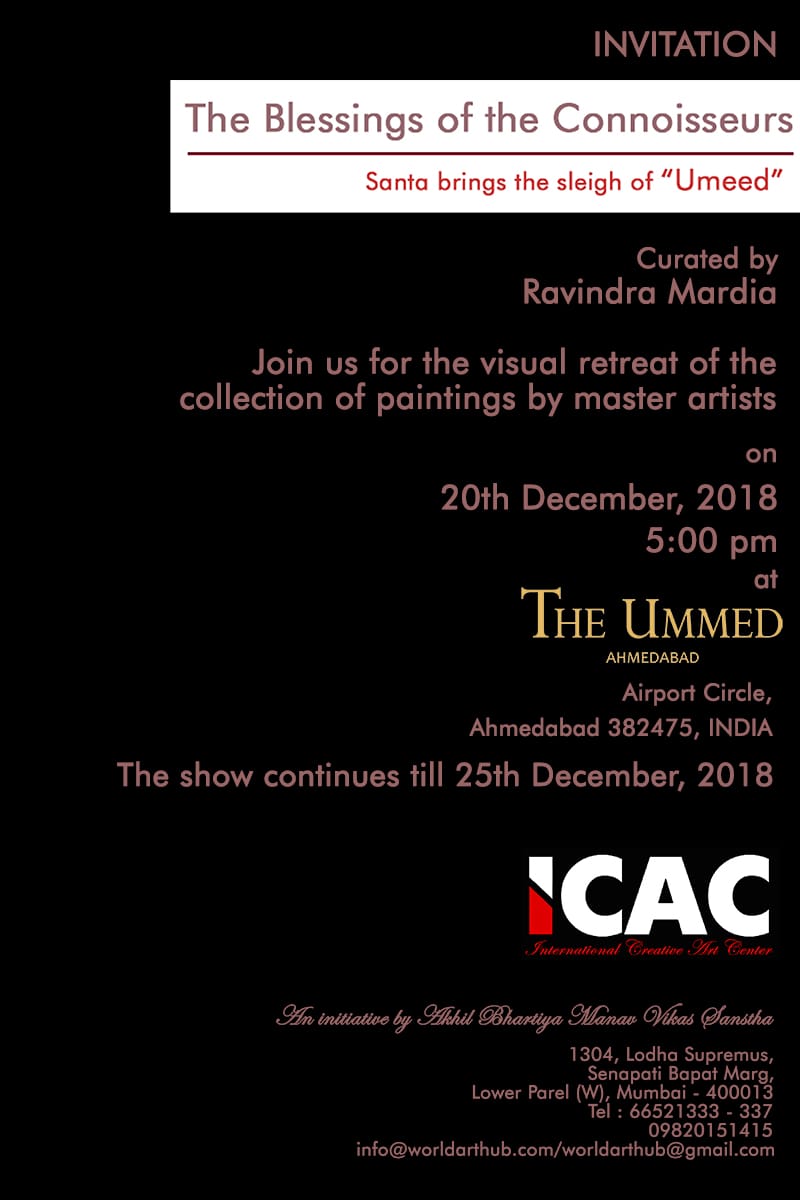The image depicts a predominantly black invitation poster, accented with white and light grey text, and featuring elements in red and purple. At the top of the invitation, the word "INVITATION" is prominently displayed, followed by the phrase "The Blessings of the Connoisseurs." In a red text beneath, it reads "Santa brings a sleigh of you made," curated by Ravindra Mardia. A visual retreat showcasing a Collection of Paintings by Master Artists is being announced, scheduled for 20th December 2018 at 5 PM, located at the UMED Airport Circle, Ahmedabad, 382475, India. The exhibition will continue until 25th December 2018. The invitation prominently features the logo "ICAC" in white and red capital letters. At the bottom, it mentions "The invitation by Michael Barihaya Maneet Samithani" and includes an email address for further inquiries.